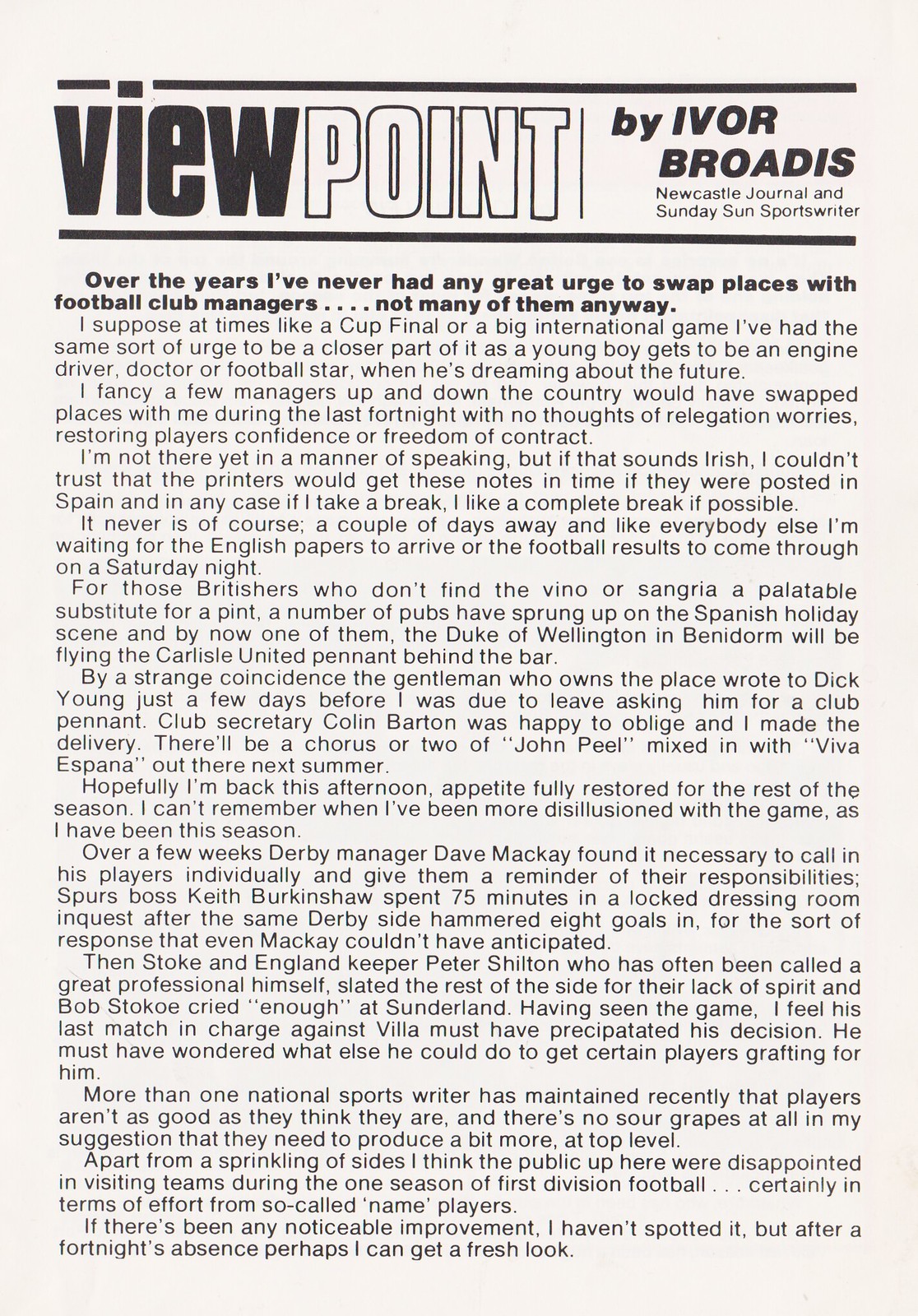The image depicts a black-and-white newspaper or magazine clipping containing a sports article titled "Viewpoint" by Ivor Brotis, a sportswriter for the Newcastle Journal and Sunday Sun. The title "Viewpoint" is visually distinct, with "View" in bold black letters on a white background and "Point" in white letters framed by black. Below the title, Ivor Brotis's byline is clearly indicated, followed by his affiliation. The article spans the full page, comprising approximately four paragraphs. In the opening lines, Ivor Brotis reflects on his lack of desire to trade places with football club managers, despite occasional moments, such as cup finals or international games, where the allure of being closer to the action tempts him. He reminisces about childhood dreams of becoming an engine driver, doctor, or football star, a sentiment he imagines is shared by others. The article likely continues to explore his observations and experiences within the world of football, including commentary on the pressures faced by managers.